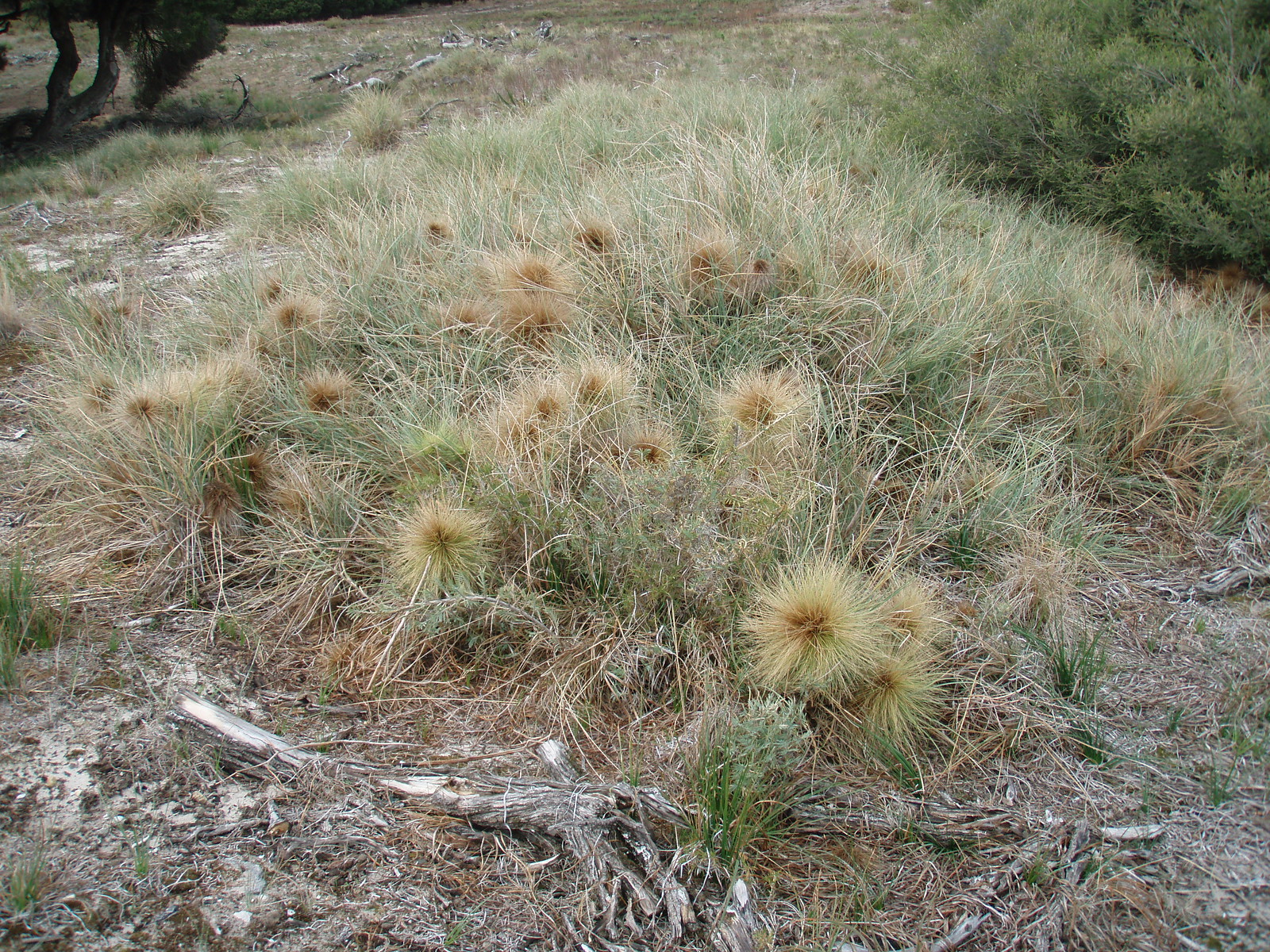This image depicts a dry, desert-like landscape taken during the daytime, but not under particularly bright sunlight. The ground, covered with a mix of dry, yellow, and green grasses, is strewn with rocks and dry twigs. Central to the image is a mound of spiky, brown, and yellowish dry grasses, likely to poke one's fingers if touched. On the top right, there is a fully green bush in stark contrast to the arid surroundings. On the top left, part of a tree trunk is visible, with branches sticking out. The background features additional foliage and the ground continuing in similar dry conditions. The scene suggests a hot climate, possibly resembling areas in Spain or South America.